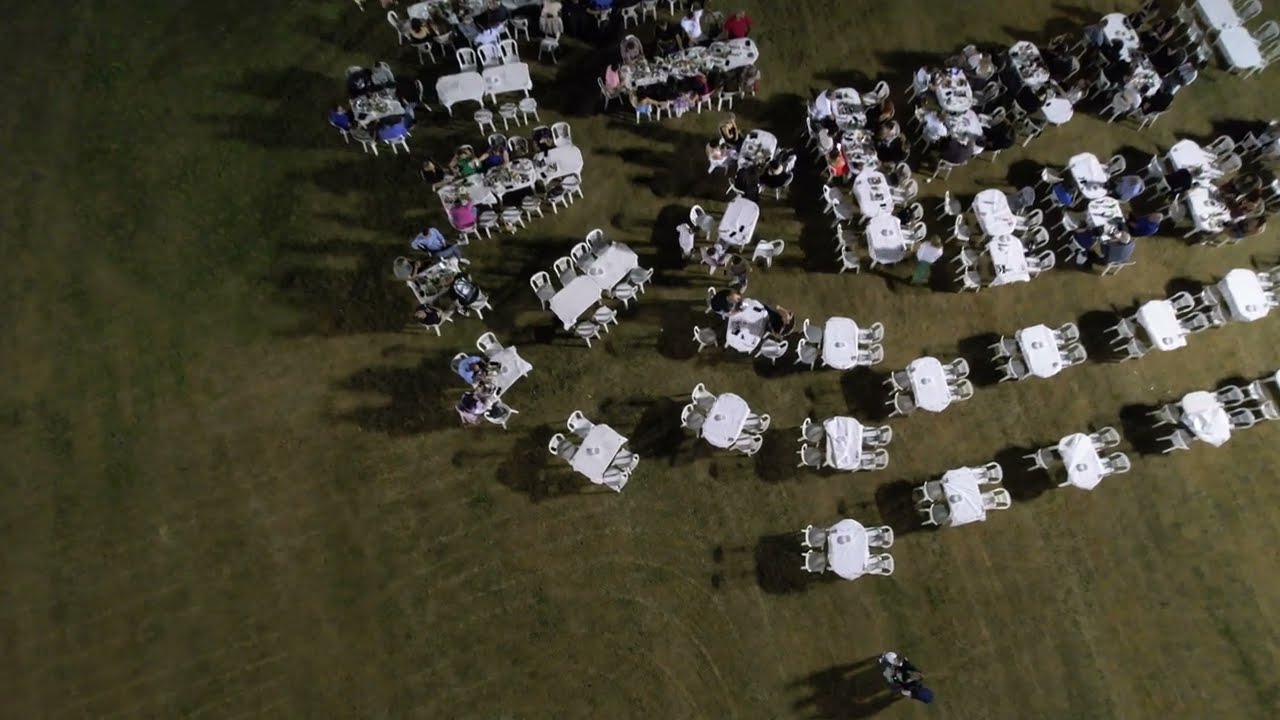This image captures an aerial perspective of a large outdoor setting, likely a wedding reception or similar event. The scene is dominated by numerous white tables draped in tablecloths and surrounded by high-back chairs. The arrangement is situated on a light green and yellow-tinted field, possibly artificial turf, or a patchy grass area. The photograph reveals a clear spatial organization: the lower rows or the first two lines of tables are vacant, while the middle and upper sections display a gradual increase in occupancy.

On closer inspection, the tables to the upper middle, right, and slightly to the left are populated by guests, identified by their colorful attire including shades of pink, blue, red, and gray. To the right, a cluster of approximately eight tables has seated guests, extending into the background where additional tables, some joined to form larger setups with around twelve seats, are partially occupied. In the upper right corner and the far back of the image, a few more tables appear unoccupied. The lighting suggests an evening or nighttime setting, with long shadows cast by artificial illumination rather than natural sunlight. This extensive view devoid of any other objects or text enhances the sense of an expansive, open-air gathering.